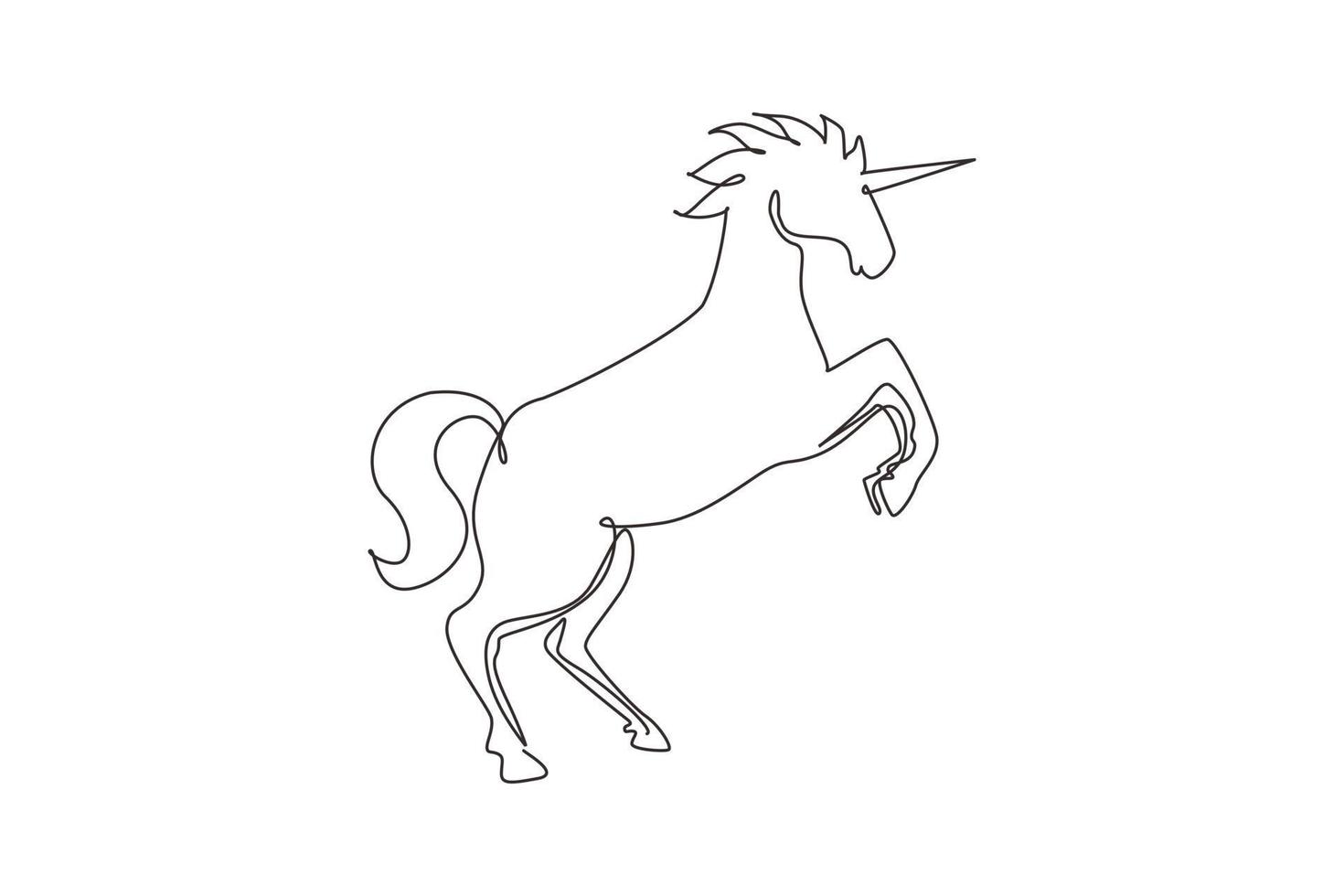The image is of a unicorn depicted in a minimalist, black-and-white, computer-generated outline, resembling a laser-printed drawing. The unicorn, standing on its two back legs, gives the impression of rearing up, with its front legs raised and parallel to each other. The horn, pointed toward the top right corner, juts prominently from the center of its forehead. The mane is stylized into six interconnected triangles, each transitioning to the next with a looping line instead of sharp points. The tail arcs in an S-shape, slightly slanted to the left. The simplistic and borderless design suggests it could be from a children's coloring book, rendered in pen or marker.